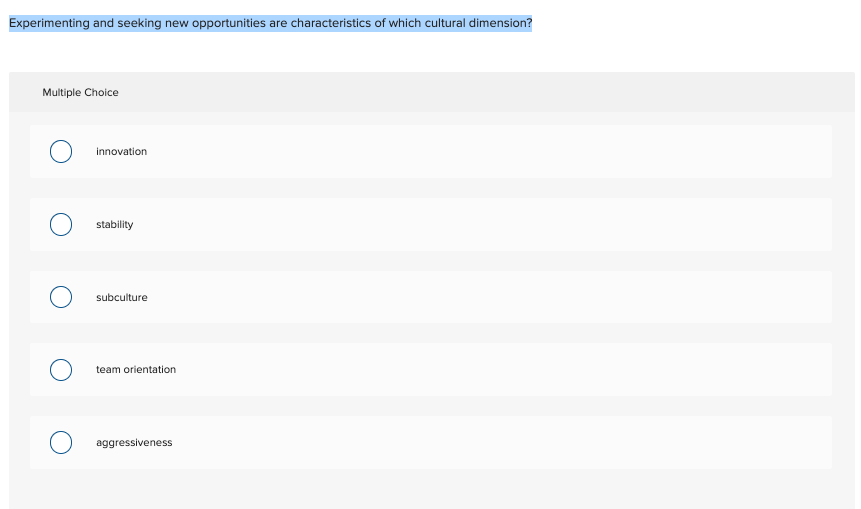The image depicts a quiz question page with a highlighted query in blue, asking, "Experimenting and seeking new opportunities are characteristics of which cultural dimension?" The text of the question is in black. Beneath the question, there are five multiple-choice options, each accompanied by a circular icon:

1. **Innovation** - represented by an empty circle.
2. **Stability** - indicated by an empty circle with a blue outline.
3. **Subculture** - also featuring an empty circle with a blue outer ring.
4. **Team Orientation** - marked by an empty circle with a blue exterior.
5. **Aggressiveness** - denoted by an empty circle with a blue border.

All the options are laid out in evenly spaced rows on a gray and white background, simulating the appearance of an online quiz interface. The options are contained within white text boxes, and the text itself is in black. The overall layout occupies the entire image, giving it a structured and digital learning platform feel.